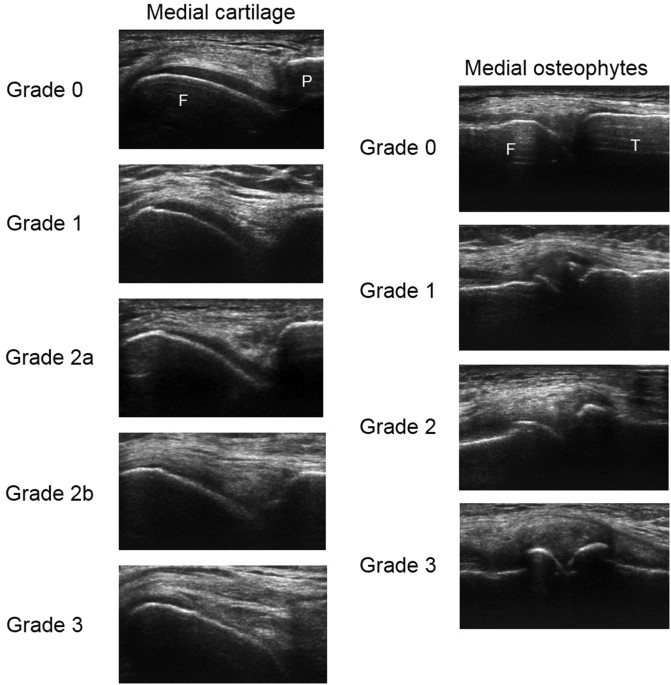The image showcases a series of ultrasound scans organized into two columns and two rows within a medical context. The first column, labeled "Medial Cartilage," contains five grayscale ultrasound images, each displaying different grades: grade 0, grade 1, grade 2A, grade 2B, and grade 3. The second column is labeled "Medial Osteophytes" and consists of four grayscale ultrasound images, labeled grade 0, grade 1, grade 2, and grade 3. All images exhibit typical black, gray, and white streaks characteristic of ultrasound imaging, with visible lines and contours that resemble hills or bumps. The precise body part remains indiscernible, though the images focus on the medial aspects of cartilage and osteophytes, highlighting their varying grades and detailed structural features.